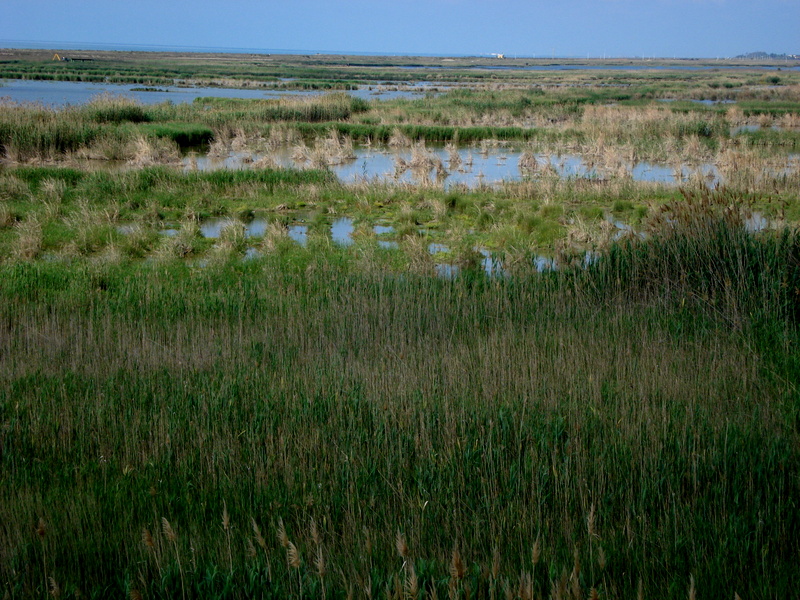This detailed photograph captures a marshy or swampy area with a blend of grassy vegetation and standing water, extending vertically through the image. The grass is a mix of green and light brown, interspersed with patches of water, creating a textured, alternating pattern. In the distance, the scene features additional swampy terrain, with structures appearing to be houses or businesses far off in the background. A tractor is visible on the left side, adding a touch of human activity to the natural landscape. A fence line and distant mountains are discernible against a clear blue sky, enhancing the depth and breadth of the scene. The photograph, taken during daytime, showcases a serene yet intricate environmental tableau, emphasizing the interplay between land and water in a marshland or lagoon setting.